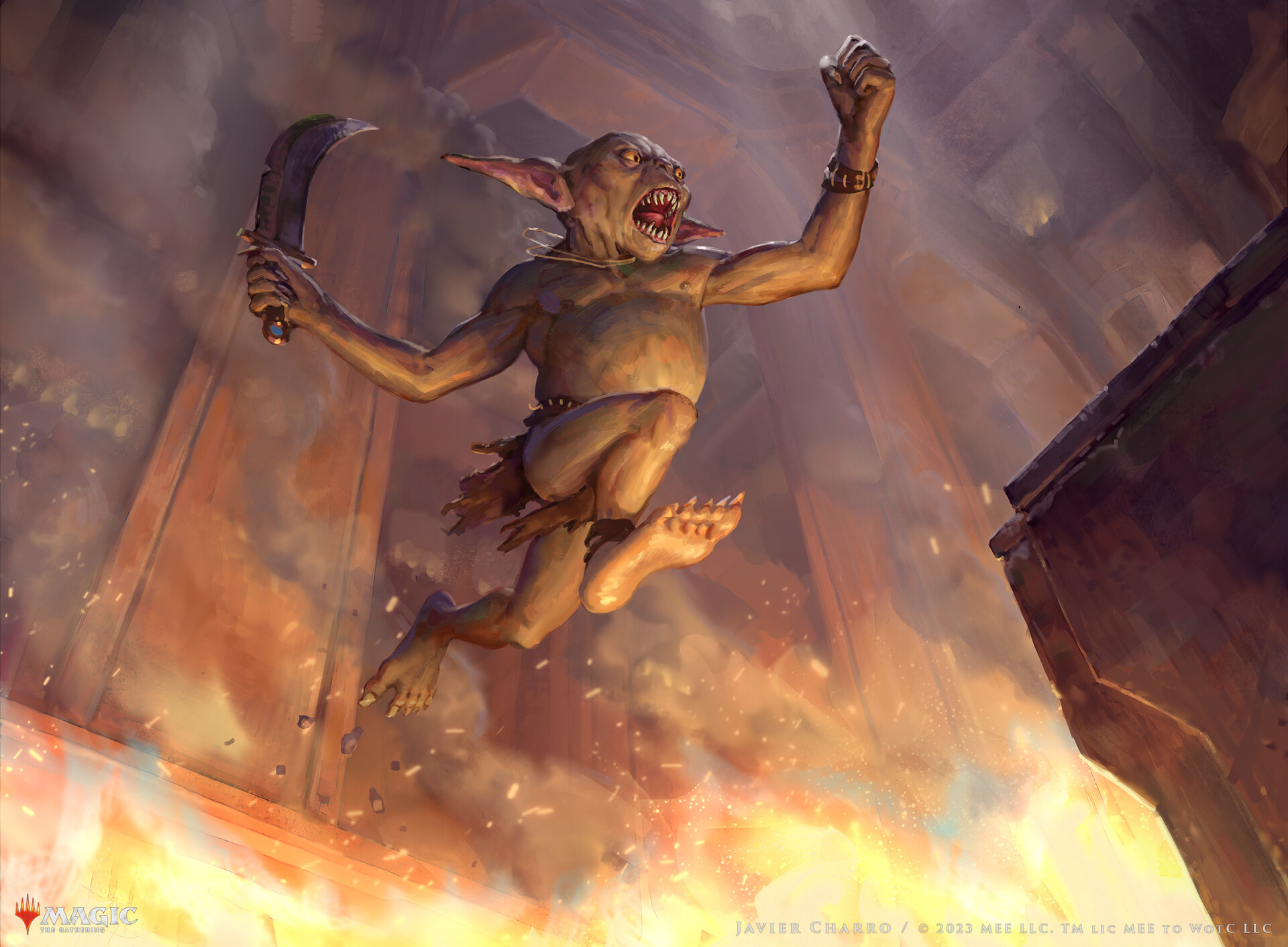The image is a detailed, multi-colored artistic piece resembling a still frame from a video game or a movie scene. It depicts a grotesque, greenish-tinted troll or ogre with long, thin pointy ears, sharp fangs, and large yellow eyes. The creature is wearing only a brown loincloth and various necklaces and bracelets. In its right hand, the troll brandishes a curved dagger or sword, and it appears to be mid-scream, baring its nasty teeth. The scene captures the troll leaping from one stone ledge to another over a massive pit of fire, with smoke and embers rising from the flames below. Surrounding the troll are grand stone structures with tall archways, suggesting a cathedral-like indoor setting lit by natural light. The image includes faint text at the bottom right corner, partially legible as "Javier Charo / 2022 M-E-E-L-L-C / TM," and features rich colors including black, white, gray, purple, orange, red, yellow, brown, silver, and pink.